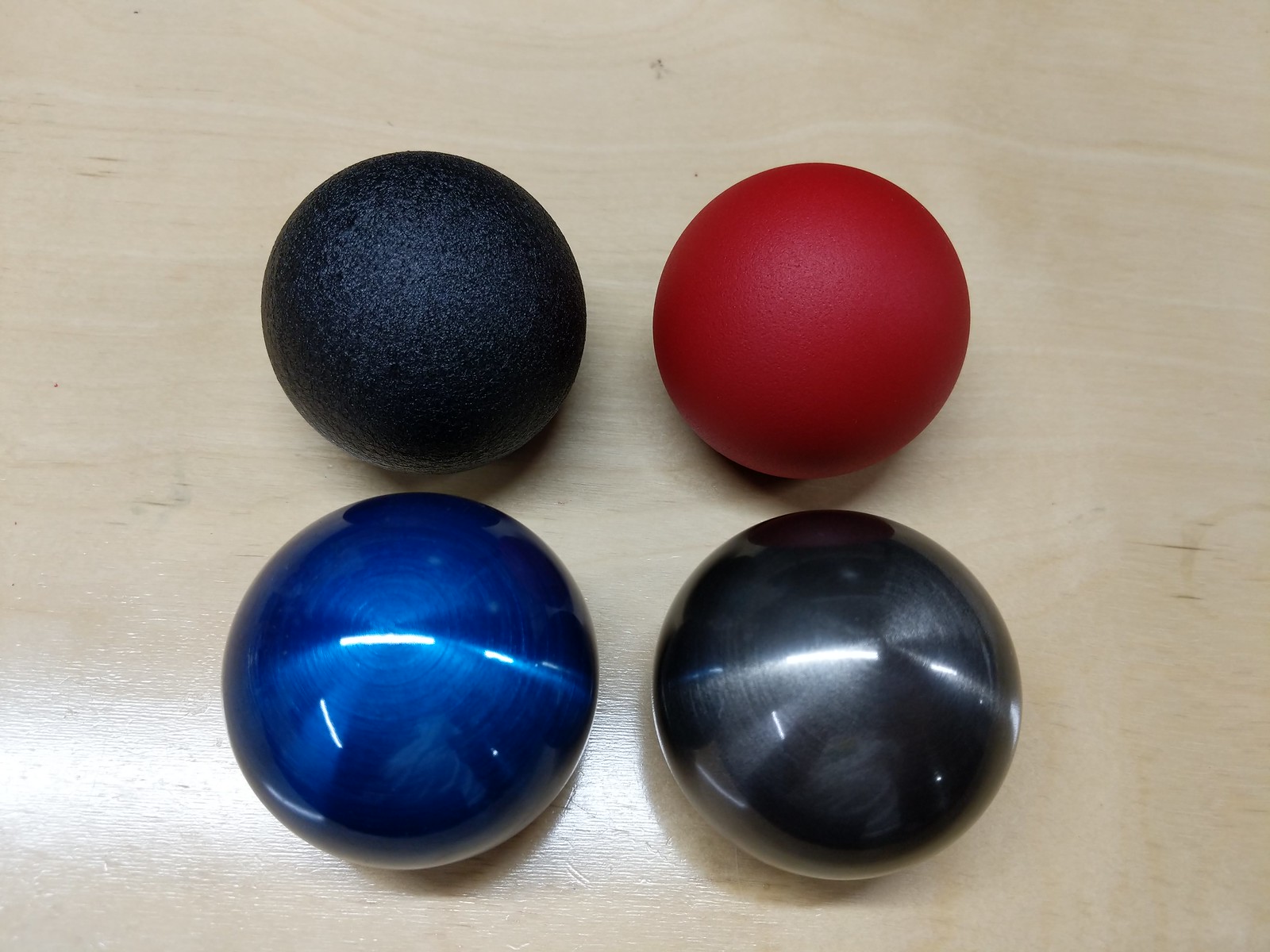The image showcases a close-up view of four round objects, arranged in a square formation, on a slightly shiny light brown wooden surface that could resemble a bowling alley floor. The top two balls are textured and evoke the appearance of dodgeballs from childhood—one black and one red. In contrast, the bottom two balls possess a smooth, glossy surface with a finish reminiscent of car paint or Christmas ornaments; one is a bright blue, and the other is a shiny gray, almost black. Each ball reflects the lighting from above, creating white splotchy highlights on their surfaces and subtle shadows on the floor. The scene is well-lit, with the light causing a distinct sheen on the balls and floor, enhancing their vibrant and contrasting textures and colors.